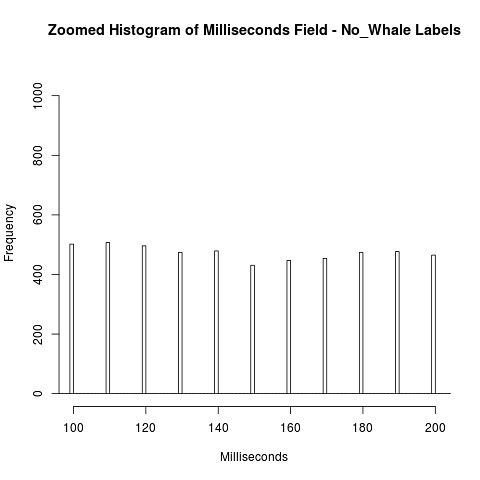The image is a detailed black and white bar graph titled "Zoomed Histogram of Milliseconds Field with No Whale Labels." The horizontal axis at the bottom represents milliseconds, ranging from 100 to 200 in increments of 20 (100, 120, 140, 160, 180, 200), while the vertical axis on the left denotes frequency, starting from 0 and increasing in increments of 200 up to 1,000. The graph features evenly spaced, hollow blue bars that indicate the frequency distribution across these millisecond intervals. Despite the uniformity in the bars' lengths, the overall presentation appears complex and challenging to interpret at a glance.